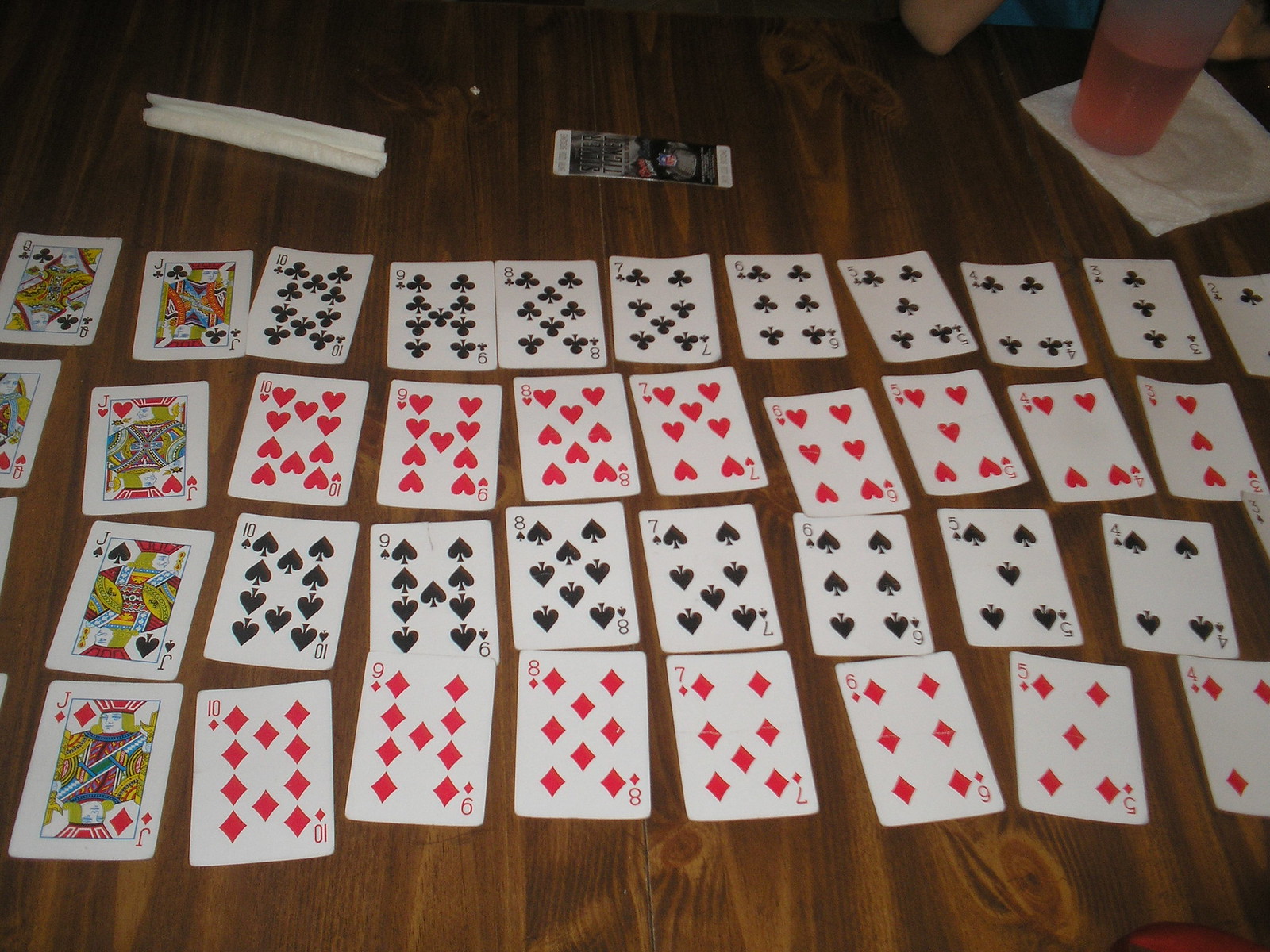The image depicts a meticulously arranged display of playing cards on a dark wooden floor. There are four rows of cards, each dedicated to one suit: the first row consists of clubs, the second of hearts, the third of spades, and the fourth of diamonds. Each row is laid out in descending order from left to right, featuring cards from Ace to King. While all 52 cards are present, only a few are distinctly visible. In the lower right corner, near the array of cards, there is a silver ticket, possibly for a sports event. Adjacent to the ticket is a rolled-up napkin. Additionally, a red plastic cup, filled halfway with water, rests atop another napkin, completing the scene.